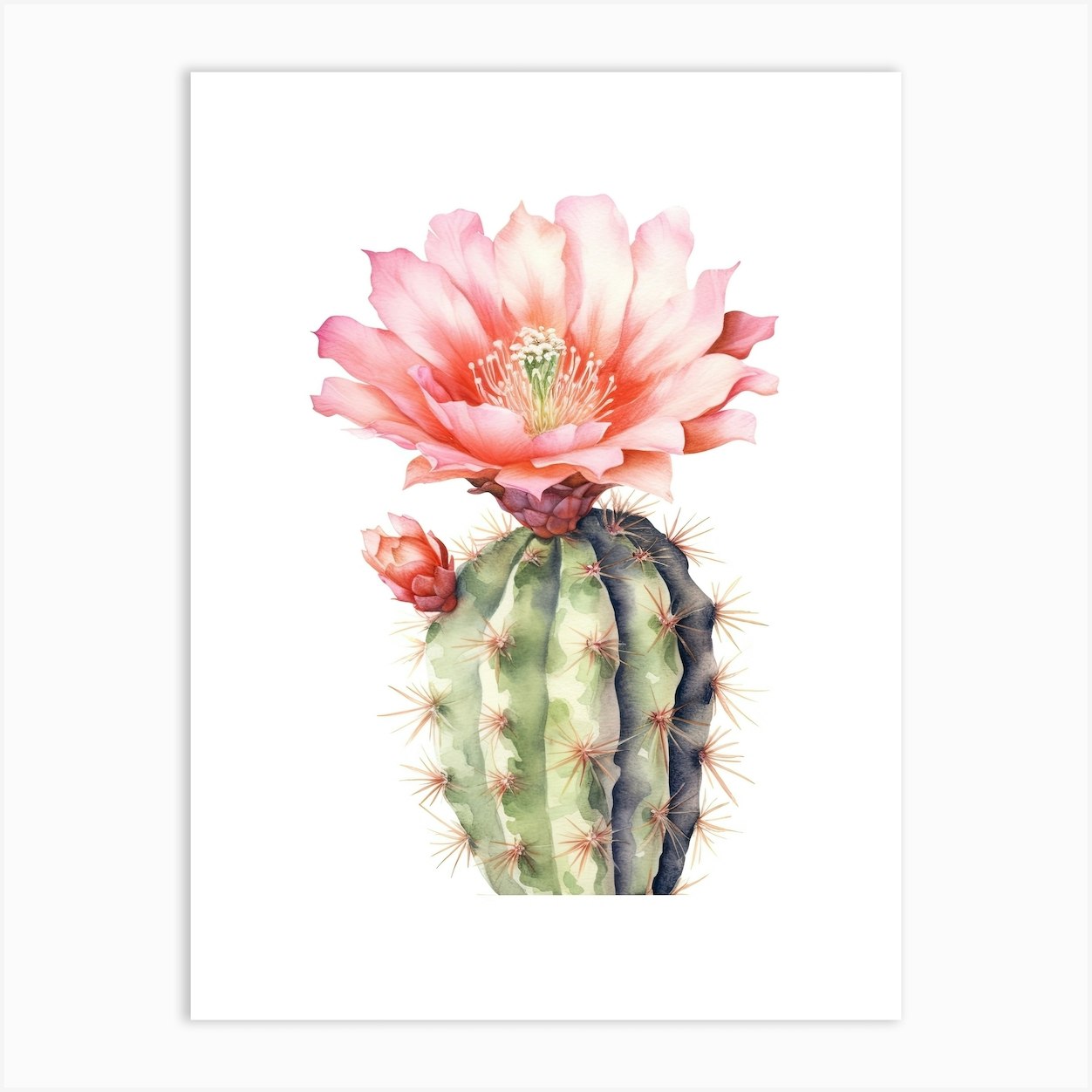The artwork is a watercolor depiction of a vibrant green cactus set against a pristine white background, encased within a white border. The cactus features numerous spikes that exhibit a gradient of colors ranging from brownish-orange to pink. Two distinct flowers adorn the cactus: a small, closed pink bud on its left side and a prominent, large bloom at the top. This grand flower is intensely pink with an intricate array of petals and delicate white stamens at its core. Accentuating its lively appearance are hints of coral and green within the flower's center. The image possesses an artificial shadow on the upper and left sides, giving it a stock photo quality, yet retaining a touch of traditional watercolor aesthetics.